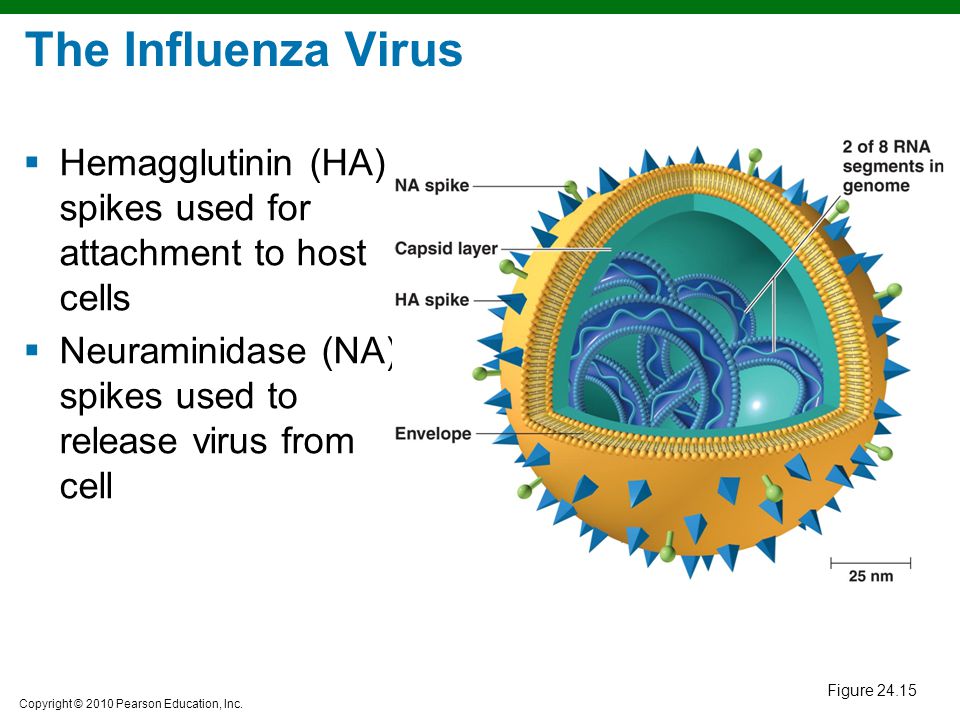### The Influenza Virus

This detailed illustration showcases the structure of the influenza virus. The title "The Influenza Virus" appears in blue beneath a prominent green bar. Below the title, two bullet points highlight key information: 
1. Hemagglutinin (HA) spikes, which are used for attachment to host cells.
2. Neuraminidase (NA) spikes, which assist in releasing the virus from the cell.

To the right of the text, there is a depiction of the influenza virus, represented as a yellow sphere with a quarter section cut out to reveal its interior. The exterior surface of the virus is adorned with numerous spikes: blue HA spikes and green NA spikes. The HA spikes are triangular and pointy, while the NA spikes have a rounded edge.

Further detailing the virus structure, the interior green lining is identified as the capsid layer, and the yellow outer shell is labeled as the envelope. Inside, blue circles with empty centers and curved lines indicate two of the eight RNA segments of the viral genome.

The illustration also includes a scale marker indicating a length of 25 nanometers (nm), providing a sense of the virus's size.